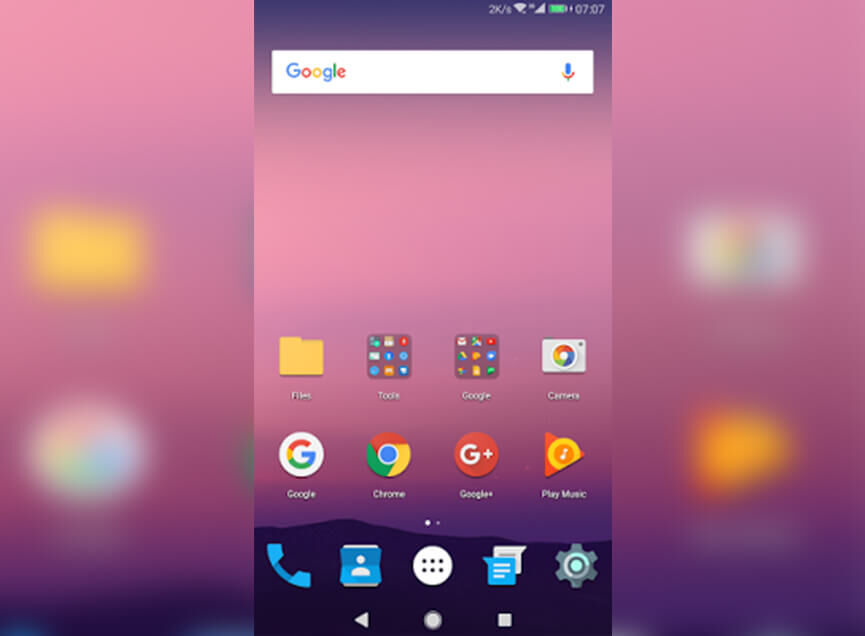The image is a horizontally oriented (landscape) screenshot, with a central focus on a vertical mobile screenshot, implying a portrait orientation within the main rectangular layout. 

The background is subtly out of focus, presenting a medium light purple hue. Within this blurred backdrop, one can discern indistinct icons including a yellow-gray icon, a blue icon to the left, and a blue-orange icon to the right, all contributing to a somewhat soft and muted visual ambiance.

The vertical mobile screenshot at the center of the image was captured at 7:07 with the battery icon showcasing a healthy green, indicating a high charge level. At the top of this screenshot, there is a white search box featuring the Google logo on the left side and a microphone icon in Google colors on the right. The background of the mobile screen exhibits a gradient purple theme, transitioning from a darker purple at the top to a dark purple silhouette resembling a mountain range towards the bottom.

Below the search bar are multiple app icons arranged in a tidy grid of three rows, each containing four or five icons. The top rows include icons for files, a couple of screenshots, Gmail, Google Chrome, Google Plus, and Play Music. The bottom row showcases essential or frequently used apps such as Phone, Contacts, Texting, and Settings, reflecting a classic and functional layout typical for a mobile device's home screen.